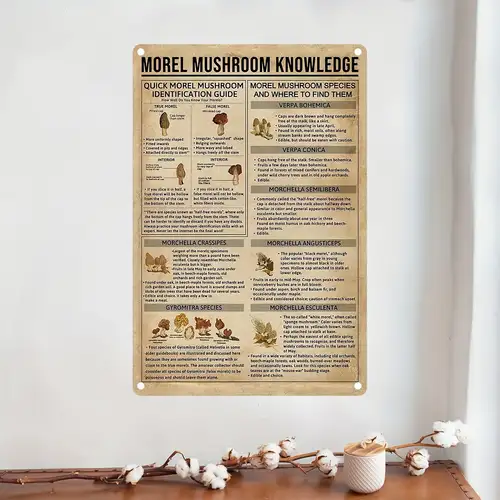This is a square image of a poster hung on a light gray or off-white wall. The poster, reminiscent of a weathered, tan-colored wanted poster, is titled in bold, uppercase black lettering: "MORAL MUSHROOM KNOWLEDGE," with an underline beneath the title. The poster is sectioned into various parts. The top left section is headed "QUICK MORAL MUSHROOM IDENTIFICATION GUIDE," displaying several images of mushrooms accompanied by descriptive text. The top right section is titled "MORAL MUSHROOM SPECIES AND WHERE TO FIND THEM," containing images and text with subheadings elaborating on different species and their habitats. The poster is affixed to the wall with four white thumbtacks, one at each corner. Below the poster is a brown wooden surface, either a tabletop or the top of a dresser, adorned with decorative twigs featuring white cotton-like balls on their stems. Additionally, there is a white, textured candle and a jar with a wooden lid placed on the surface.